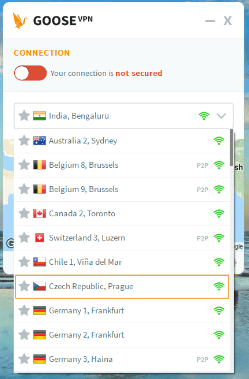The image showcases a dual-layered pop-up interface. The foremost pop-up features a list of servers with respective locations and connection statuses. Each entry is formatted with a gray star icon on the left, followed by a country's flag, country name, city name, and a green Wi-Fi signal indicator on the right. Detailed entries include:

1. A gray star with the Indian flag labeled "India, Bangalore."
2. A gray star with the Australian flag labeled "Australia, Gamma, Sydney."
3. A Belgian flag labeled "Belgium, Eight, Brussels."
4. Another Belgian flag labeled "Belgium, Nine, Brussels."
5. A Canadian flag labeled "Canada, Two, Toronto."
6. A Swiss flag labeled "Switzerland, Three, Luzern."
7. A Chilean flag labeled "Chile, One, Villavademar."
8. A Czech flag labeled "Czech Republic, Prague" with an orange box highlighting it.
9. A German flag labeled "Germany, One, Frankfurt."
10. Another German flag labeled "Germany, Two, Frankfurt."
11. A third German flag labeled "Germany, Three, Haina."

The overlaying pop-up is partially obscured, showing "Goose VPN" in black at the top, followed by an orange box with "Connection" within, and a red "Your connection is not secure" warning. In the background, parts of a map are visible, with green and blue hues on the right side and beige and blue hues on the left.